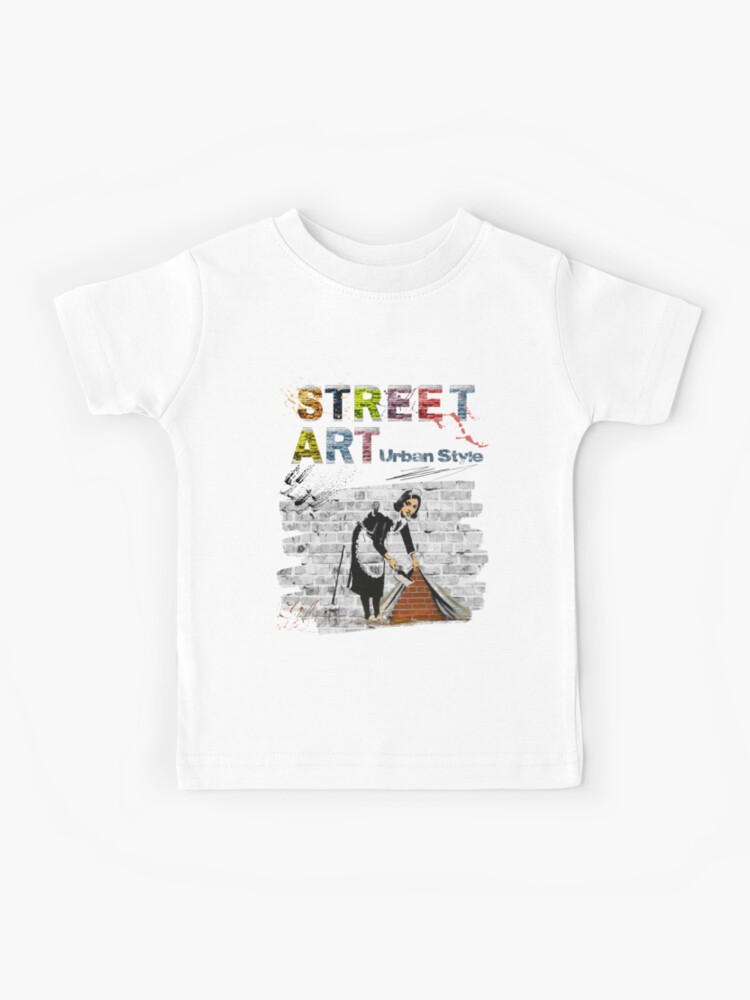The image depicts a vertically oriented photograph of a white, short-sleeved cotton t-shirt with a slightly darker, rounded neckline. Laid flat to reveal its front, the t-shirt features a bold, colorful design. At the top, the text "STREET ART" is prominently displayed with each letter in a different vibrant color—S (orange), T (red/blue), R (green/yellow), E (purple), and T/A/T (pink/blue/red). Below this, in smaller blue print, is the phrase "URBAN STYLE." Underneath the text, a detailed illustration occupies the central part of the t-shirt. The illustration shows a woman in a black maid outfit, complete with an apron and hairpiece. She stands in front of a gray brick wall, lifting a section of it as if it were a cloth, to reveal a brown brick wall beneath. The image suggests a scene where the woman is exposing a hidden reality behind the superficial facade of the gray wall.